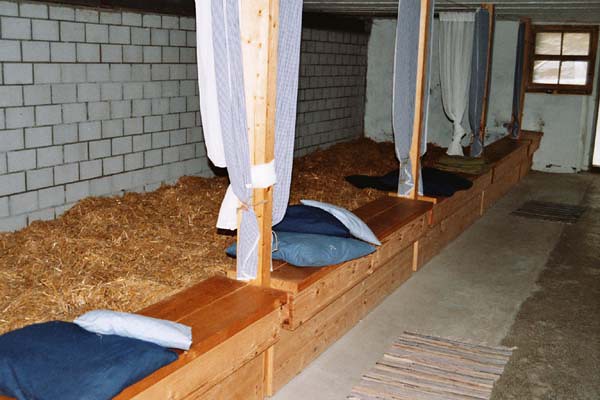This image depicts an interior setting, possibly a makeshift shelter or rudimentary living space, characterized by a white brick or cement back wall. In front of the wall is a layer of yellowish-brown hay, encircled by vertical wooden poles that create distinct, curtained-off sections, perhaps designed for sleeping or privacy. Each section houses blue and white pillows, some appearing homemade from blue fabric, placed on a dark brown bench with wooden panels beneath it. The floor is a mix of light and dark concrete, adorned with two throw rugs for added comfort, one of which features vertical stripes. A brown window frame with crisscrossing elements and glass panes completes the background, suggesting a rustic and improvised environment.